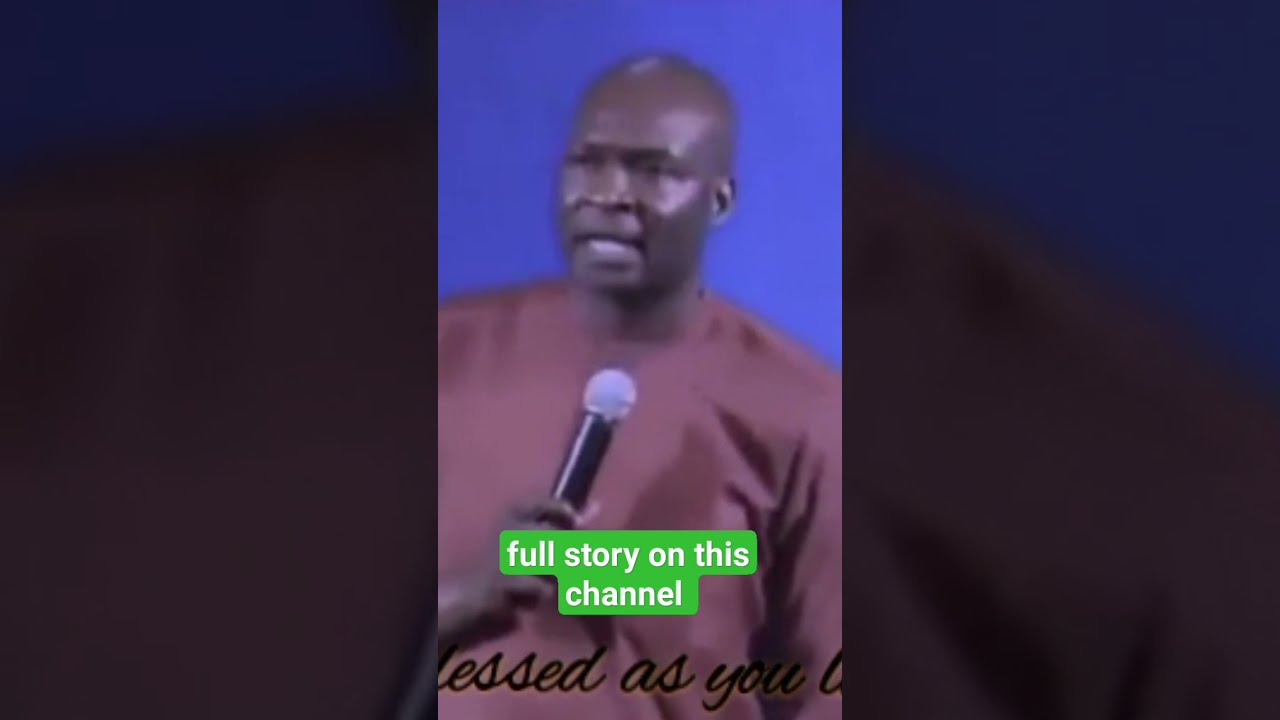In a slightly blurry image, a bald black man, possibly in his 50s or 60s, is seen holding a typical black microphone with a gray top close to his mouth, which is partially open as if he is speaking. He appears to have a serious or stern expression on his face. The man is dressed in a long-sleeved reddish-orange sweatshirt and is positioned against a blue background. His right hand grips the microphone at about chest height, covering part of his hand. There is noticeable shine on his forehead and cheeks, giving him a bit of a round face but not an overweight appearance. Along the bottom of the image, in white cursive writing on a green background, are the partially cut-off words "blessed as you," followed by some illegible text. The text "full story on this channel" is also prominently displayed in white letters against a green background.